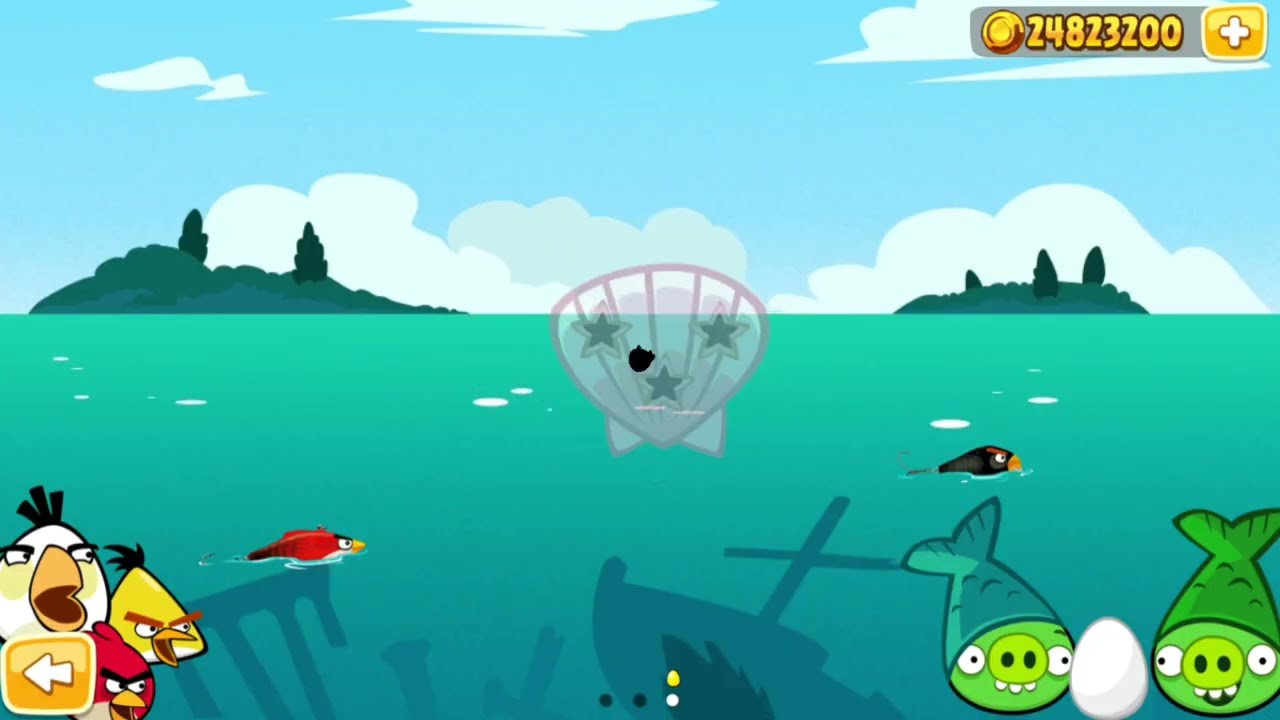This image is a detailed screenshot from a video game resembling Angry Birds, set in an ocean environment. The bottom half of the scene is dominated by a greenish-blue body of water with white spots, suggestive of waves or foam, and the outlines of submerged features like ship remnants and city ruins. In the bottom right corner, two green fish-like creatures with pig snouts can be seen, with a chicken egg placed between them. Meanwhile, the bottom left corner features three iconic Angry Birds characters: the red bird, the triangular yellow bird, and the large white bird, all with angry expressions. An orange square with a leftward-pointing white arrow likely represents a back button. Flanking the body of water on the left and right are lush green land masses with dark green trees, and above them stretches a light blue sky dotted with white and gray clouds, some extending beyond the horizon. Dominating the middle of the image is a semi-transparent clamshell adorned with stars. In the top right corner, the game's current score is displayed in golden coins, marked by the number 24823200 followed by a plus sign.